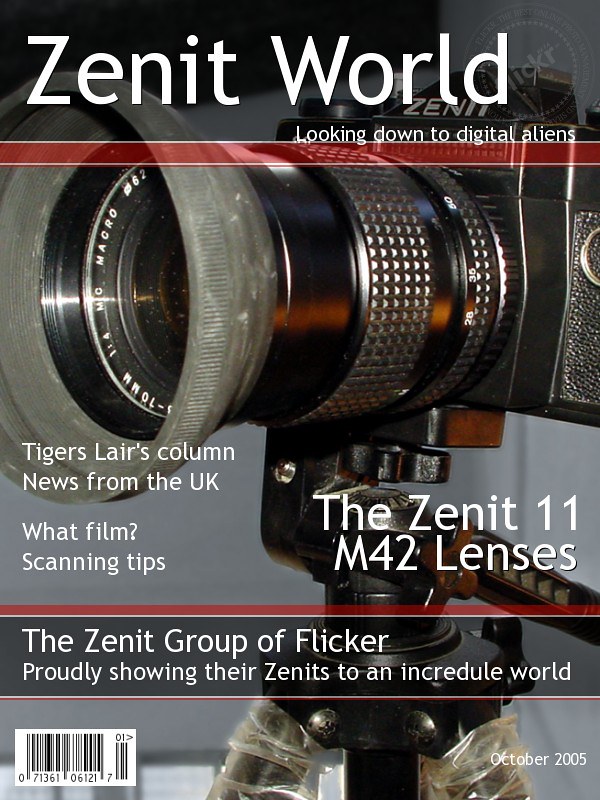The image depicts a magazine cover featuring an up-close photograph of a camera mounted on a tripod. Highlighted prominently across the top in bold, white letters is the title, "Zenit World," followed by the phrase, "Looking Down to Digital Aliens." The camera, angled slightly to the side with its lens facing forward, occupies the center of the image. On the left side of the camera, the text reads, "Tiger's Lair's Column, news from the UK, What Film Scanning Tips?" On the right side, it states, "The Zenit 11 M42 Lenses". Below the camera image, in white letters, it says, "The Zenit group of Flickr, proudly showing their Zenits to an incredible world." The bottom section of the cover features a red-bordered margin, containing a UPC code on the left and the date "October 2005" on the right. The overall background of the cover is a sophisticated grey, enhancing the sleek look of the prominently featured camera and its long lens.